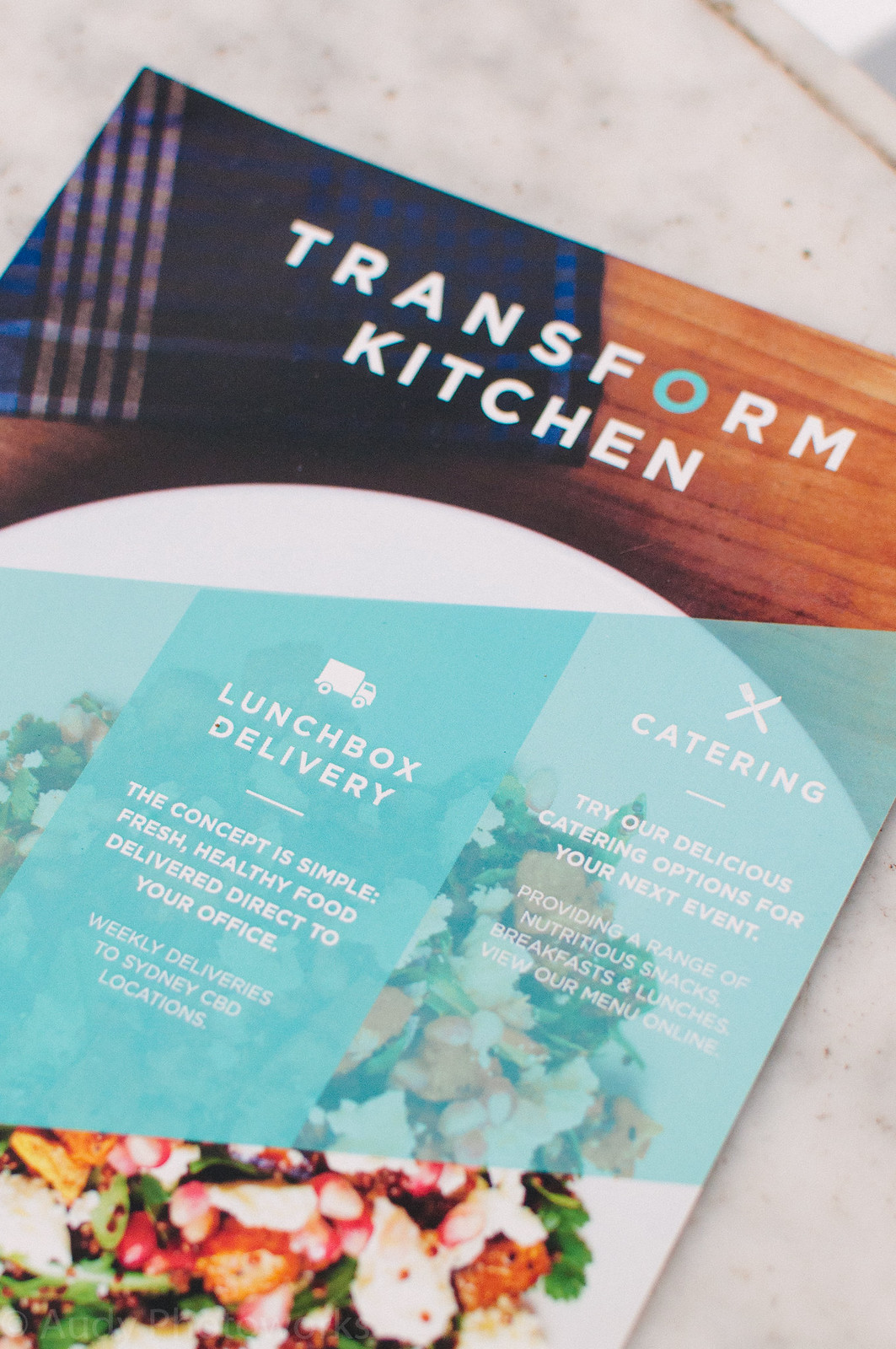This is a photo of a pamphlet titled "Transform Kitchen" set on a white granite or marble kitchen countertop. The top section of the pamphlet showcases the title against the plain backdrop. Below, a colorful section features an image of a plate of food, possibly a chicken salad. Superimposed on this image is a blue bar with the darkest part reading "Lunch Box Delivery" and a small drawing of a truck above it. The text on the blue bar states, "The concept is simple, fresh healthy food delivered direct to your office, weekly deliveries to Sydney CBD locations." To the right, in a lighter blue section, it reads "Catering" along with a picture of a knife and fork crossed above it. The catering section promotes, "Try our delicious catering options for your next event providing a range of nutritious snacks, breakfasts, and lunches. View our menu online."